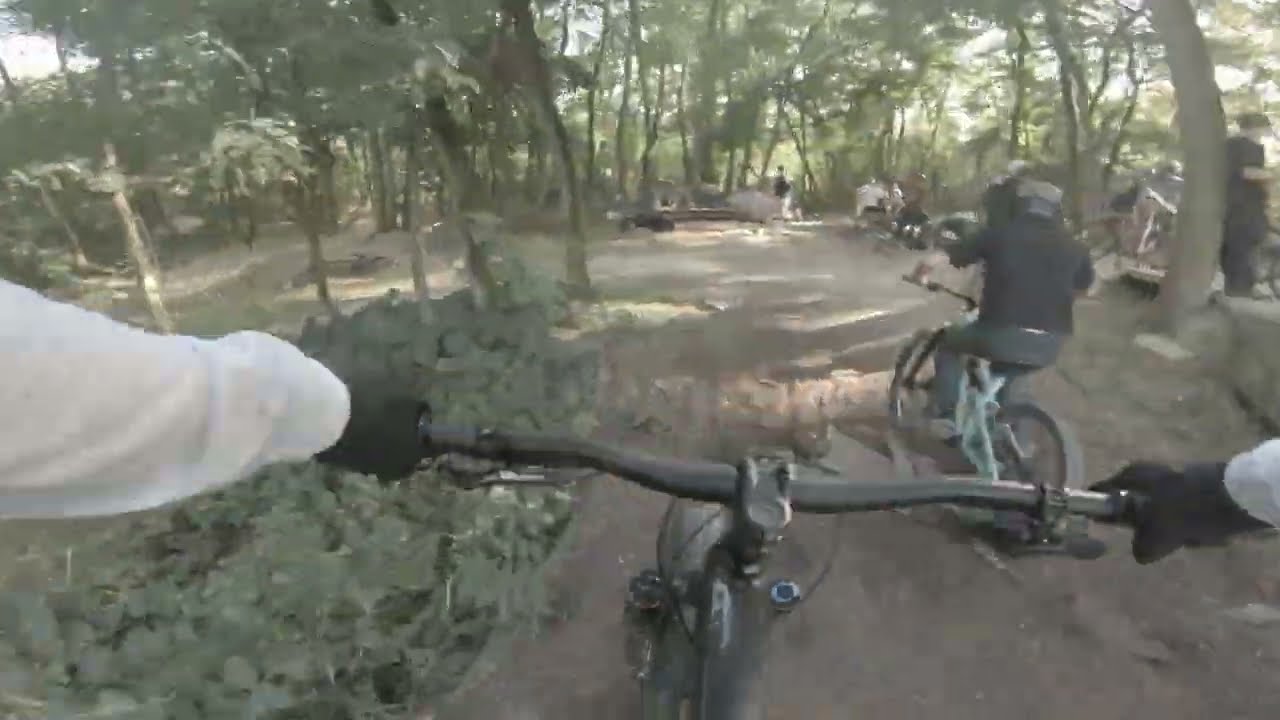The photograph, captured with a lower-quality camera that introduces a grainy texture, portrays a lively scene of mountain biking on a sunlit, dirt trail in the woods. Taken from the perspective of the person riding, the image features their arms, dressed in dark gloves, gripping the bike's handlebars. The motion creates a noticeable blur, adding a dynamic feel to the picture. To the left of the trail, there are small plants, bushes, and several tall trees, while the right side includes another rider ahead and more individuals in the distance, some of whom appear to be standing or milling around the path. Despite the blur and low clarity, the vibrant green of the foliage and the earthy tones of the dirt path are evident, suggesting a bright day with plenty of natural light filtering through the canopy.